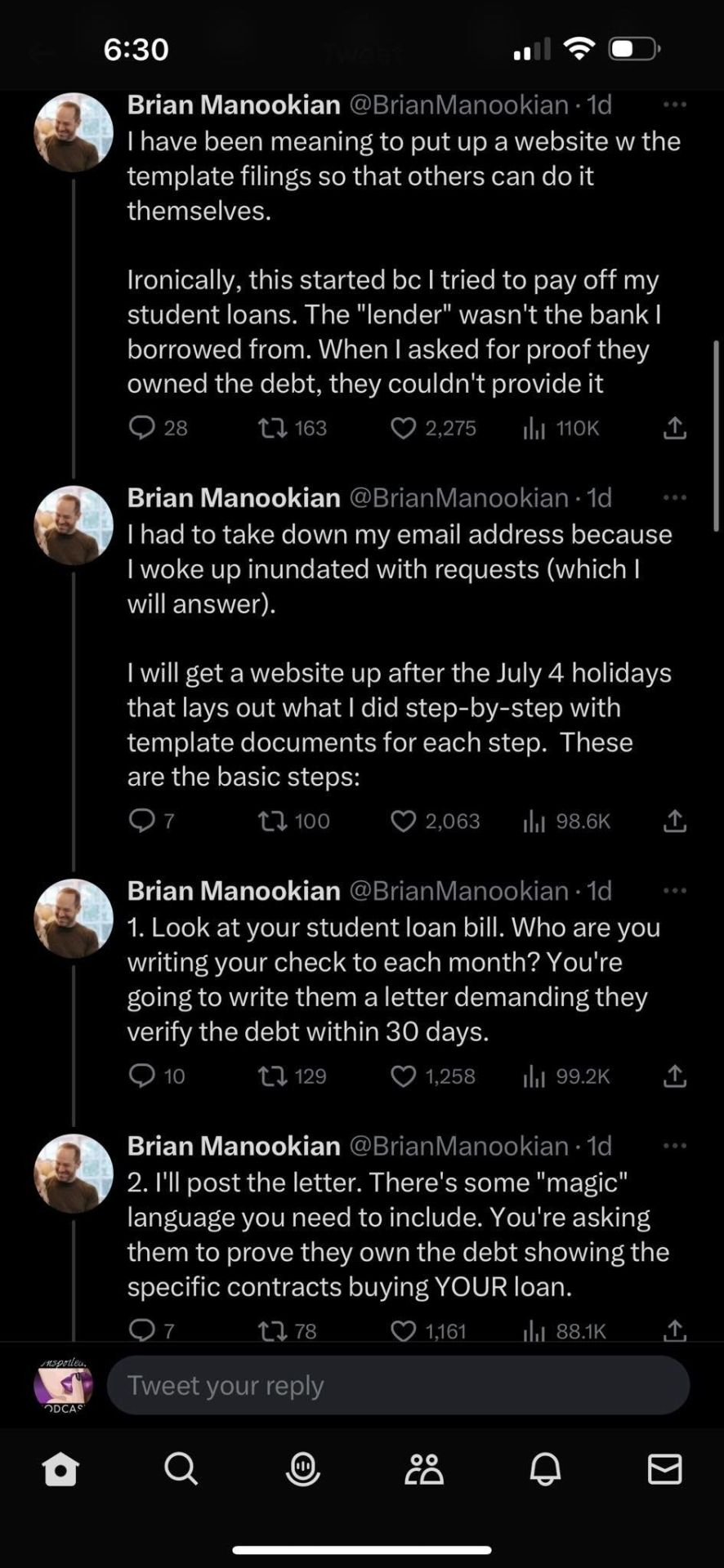This is a highly detailed screenshot of a Twitter conversation featuring multiple tweets from the same user. The interface is set to dark mode, giving the background a black appearance. 

**Top Section:** 
- **Left Corner:** The timestamp "6:30" is displayed about an inch from the left edge.
- **Right Corner:** The battery icon appears half full (white and black), alongside a fully filled Wi-Fi signal icon symbolized by two white boulders and two gray bars.

**First Tweet:**
- **Profile Picture:** Displays a man with short hair wearing a black shirt against a blue background.
- **Username:** "Brian Manookian" in bold white text, with the handle "@BrianManookianM1D" in gray, followed by three ellipsis dots.
- **Content:** Two initial lines followed by a single word, then a space, and four more lines. The tweet addresses topics like student loans, banks, and debt.
- **Icons and Metrics:** 
  - Comment Icon (28 replies)
  - Retweet Icon (163 retweets)
  - Like Icon (2,275 likes)
  - Engagement Icon (110 engagements)

**Second Tweet:**
- **Content:** Three lines of text, followed by a space, then four more lines. 
- **Icons and Metrics:**
  - Comment Icon (4 replies)
  - Retweet Icon (100 retweets)
  - Like Icon (2,063 likes)
  - Engagement Icon (98.6K views)

**Third Tweet:**
- **Content:** Starts with one dot, followed by four lines of text.
- **Icons and Metrics:**
  - Comment Icon (10 replies)
  - Retweet Icon (129 retweets)
  - Like Icon (1,256 likes)
  - Engagement Icon (99.2K views)

**Fourth Tweet:**
- **Content:** Begins with "two point," then followed by four lines of text.
- **Icons and Metrics:**
  - Comment Icon (7 replies)
  - Retweet Icon (78 retweets)
  - Like Icon (1,161 likes)
  - Engagement Icon (88.1K views)

**Navigation Bar at the Bottom:**
- A gray bar prompts the option to "Tweet your reply."
- Icons for navigation: House, Search, Microphone, Friends, Bell, and Email.
- A white line is centered at the bottom.

This thorough description encapsulates the entire layout and specific details of the Twitter thread, highlighting the repeated posts and engagement metrics by Brian Manookian.